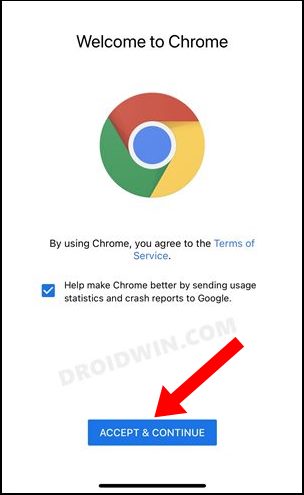The image appears to be a vertical mobile screenshot showcasing the initial landing page of the Chrome app upon first download on a smartphone device. The background is predominantly white, with "Welcome to Chrome" prominently displayed at the top in black text. Directly beneath this welcoming message is the iconic Chrome symbol, composed of a circle divided into three colorful segments resembling a pinwheel—one red third, one yellow third, and one green third. At the center of this symbol is a blue circle outlined in white.

Below the Chrome symbol, a message reads, "By using Chrome, you agree to the Terms of Service," with "Terms of Service" highlighted in blue, indicating it’s a clickable link. Further down is a blue checkbox containing a white checkmark, followed by the statement, "Help make Chrome better by sending usage statistics and crash reports to Google."

The screenshot also features a subtle gray watermark reading "droidwind.com" and a conspicuous long red arrow pointing to a rectangular blue button with white text that says, "Accept and continue." At the very bottom, there is a thin horizontal black line that spans the width of the "Accept and continue" button.